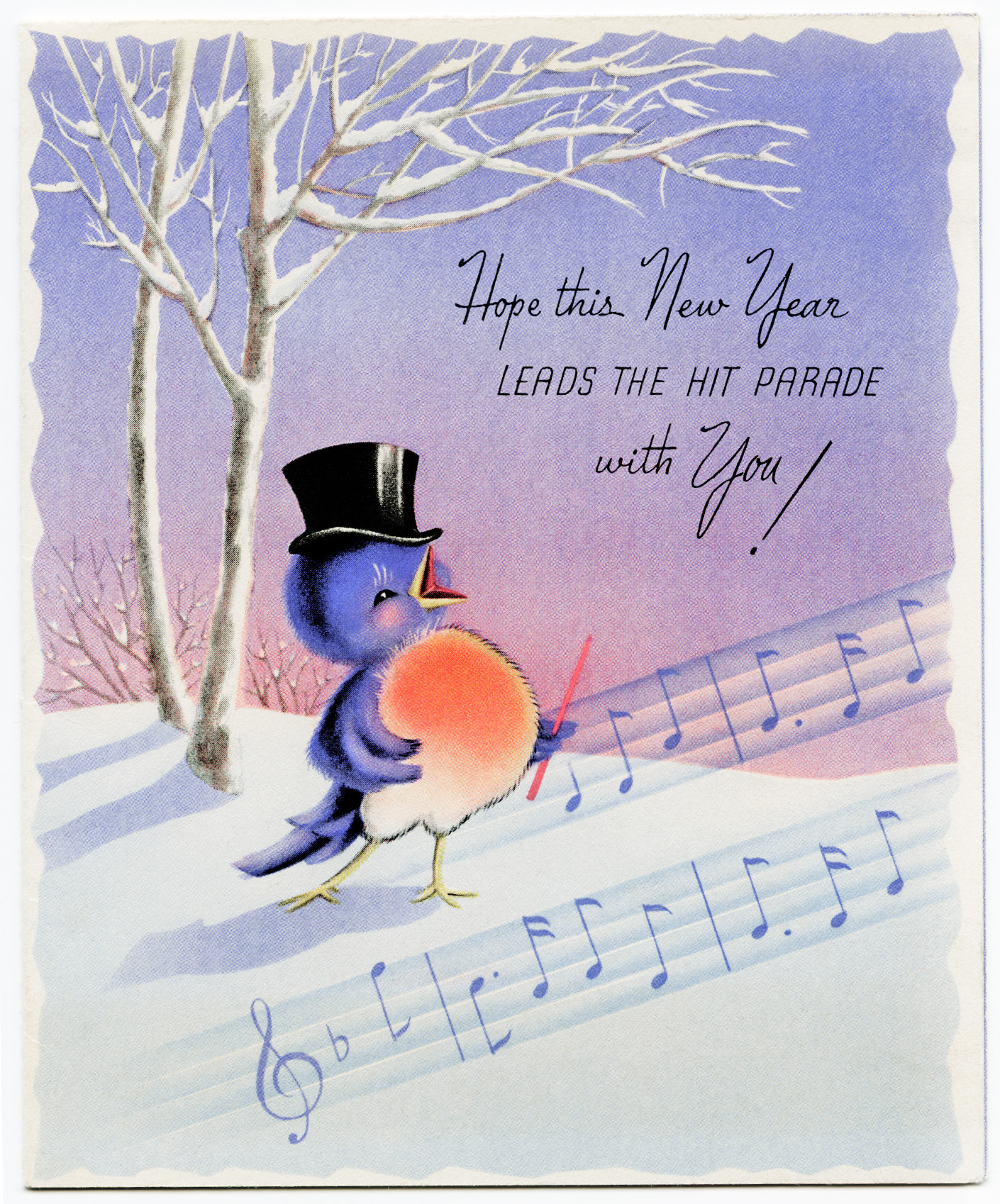This detailed and vibrant illustration on a holiday greeting card features a cheerful scene that captures the joyful spirit of the new year. The card’s outer edges are white with a scalloped pattern, framing a lively portrayal in the center. Dominating the image is a small, jubilant blue bird adorned with a black top hat and rosy cheeks. The bird has a vivid orangish chest that fades to white towards the bottom and bright yellow legs and feet. Standing on a snowy hillside, the bird is joyfully singing with its beak open wide, holding a red conductor’s baton in its left wing. Surrounding the bird are strips of sheet music and musical notes, accentuating its song. The background features a prominent bare-branched tree covered in snow, with hints of additional trees barely visible. Above the bird, in elegant black cursive text, it reads, "Hope this new year leads the hit parade with you!" This charming and vintage-inspired card captures a festive and hopeful message, perfect for celebrating the new year.